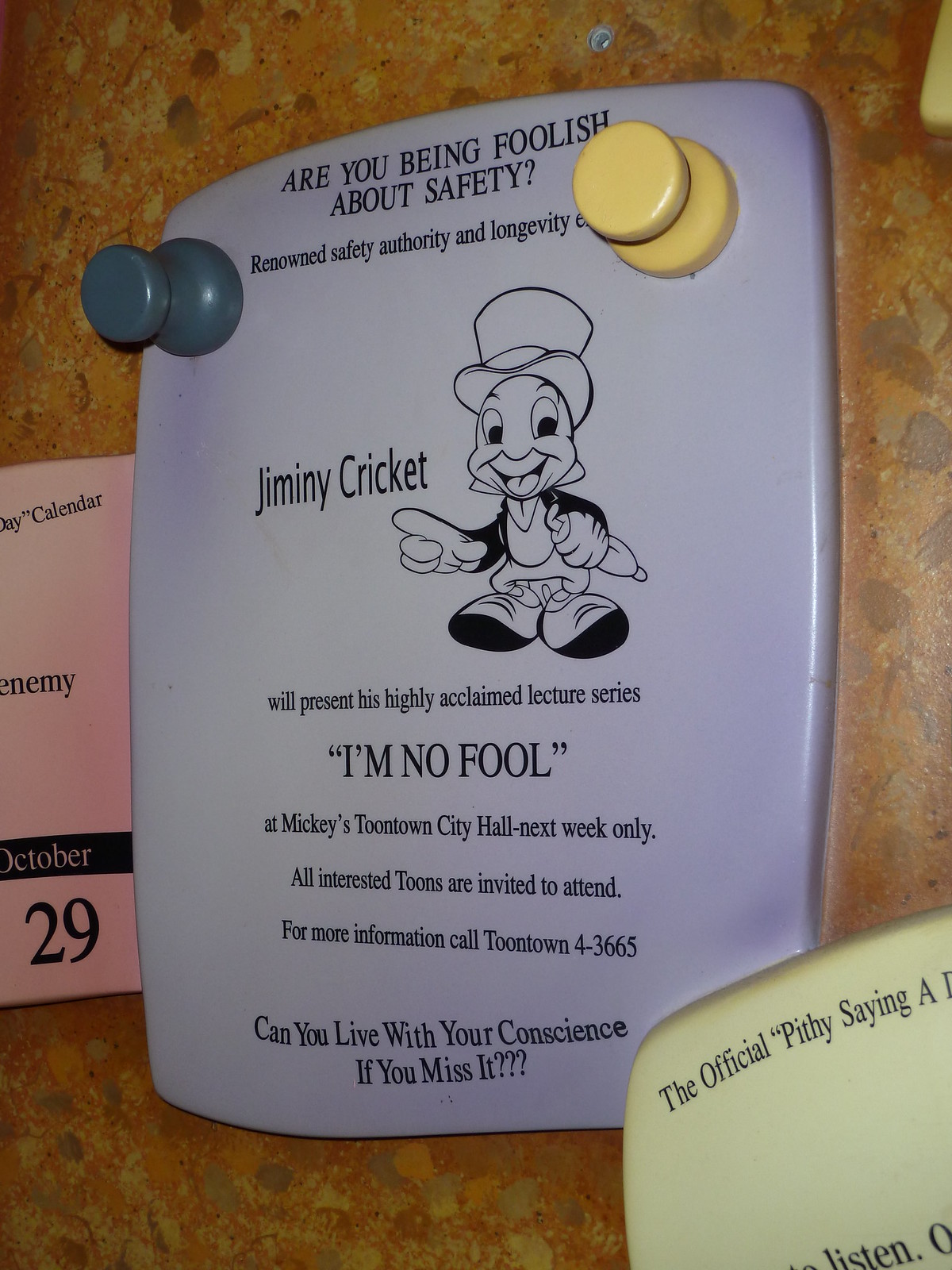This photograph captures a section of a bulletin board, possibly located in an area resembling Disneyland. The centerpiece is a rectangular, purple plaque with beveled edges, adorned with cartoonish blue and yellow pushpins on the left and right corners. The background of the bulletin board is painted brown with blotches of light brown, gray, and tan hues.

Prominently displayed on the plaque is an illustration of Jiminy Cricket, clearly labeled with his name. Surrounding the image is black text that reads: "Are you being foolish about safety? Renowned safety authority and longevity." Due to the positioning of the right pushpin, one word in the line is obscured. Below the picture of Jiminy Cricket, additional text announces: "Jiminy Cricket will present his highly acclaimed lecture series 'I Am No Fool' at Mickey's Toontown City Hall next week only. All interested Toons are invited to attend. For more information call Toontown 4-3665." The plaque concludes with the poignant question: "Can you live with your conscience if you miss it?"

Adjacent to this plaque, partially visible on the bulletin board, is a pink sign with text that includes "calendar," "enemy," and "October 29th."